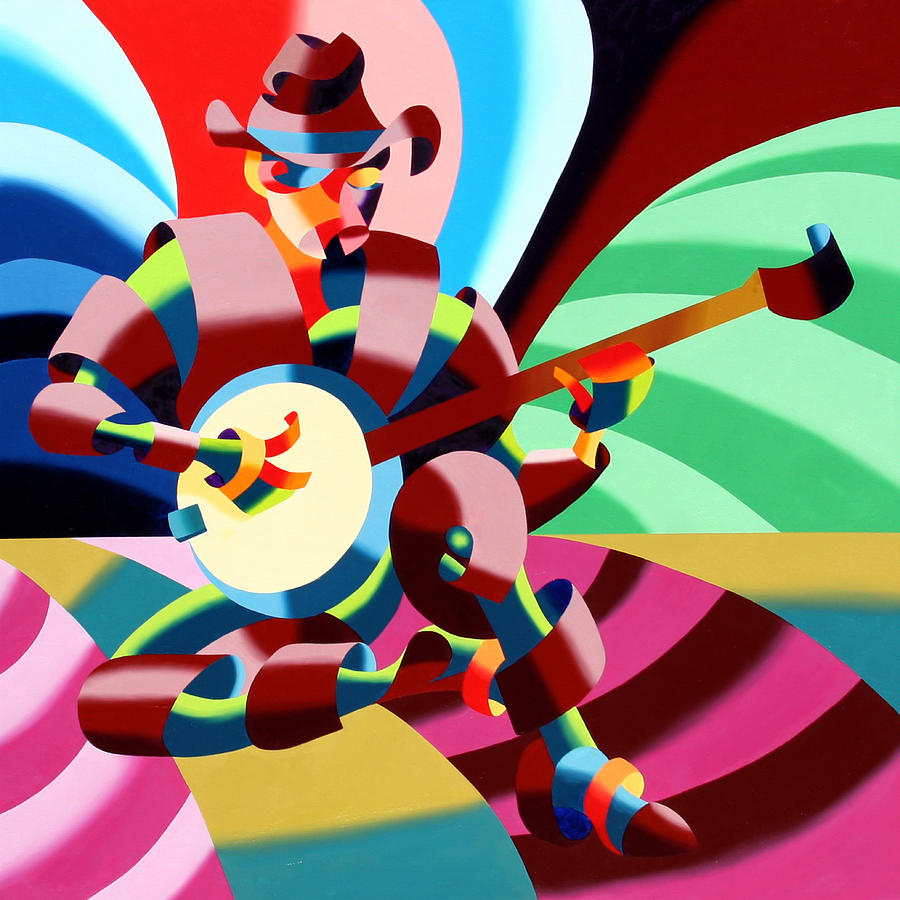The image is a highly colorful abstract painting depicting a figure playing a banjo. The figure, which appears to be a mechanical animal or a man, is adorned in a cowboy hat and is seated with one leg bent up and the other to the side. Vibrant and swirling ribbons of colors—pinks, reds, greens, lime green, maroons, blues, yellows, golds, and whites—form the image, giving it a candy cane stripe and Cheshire cat-like pattern. The figure’s skin bears a futuristic, blue and green hue, with one eye yellow and the other blue, adding to its cartoon-like, CGI appearance. The background features vivid, multi-colored designs reminiscent of zoomed-in details from the NBC peacock logo, enhancing the abstract and surreal nature of the artwork.